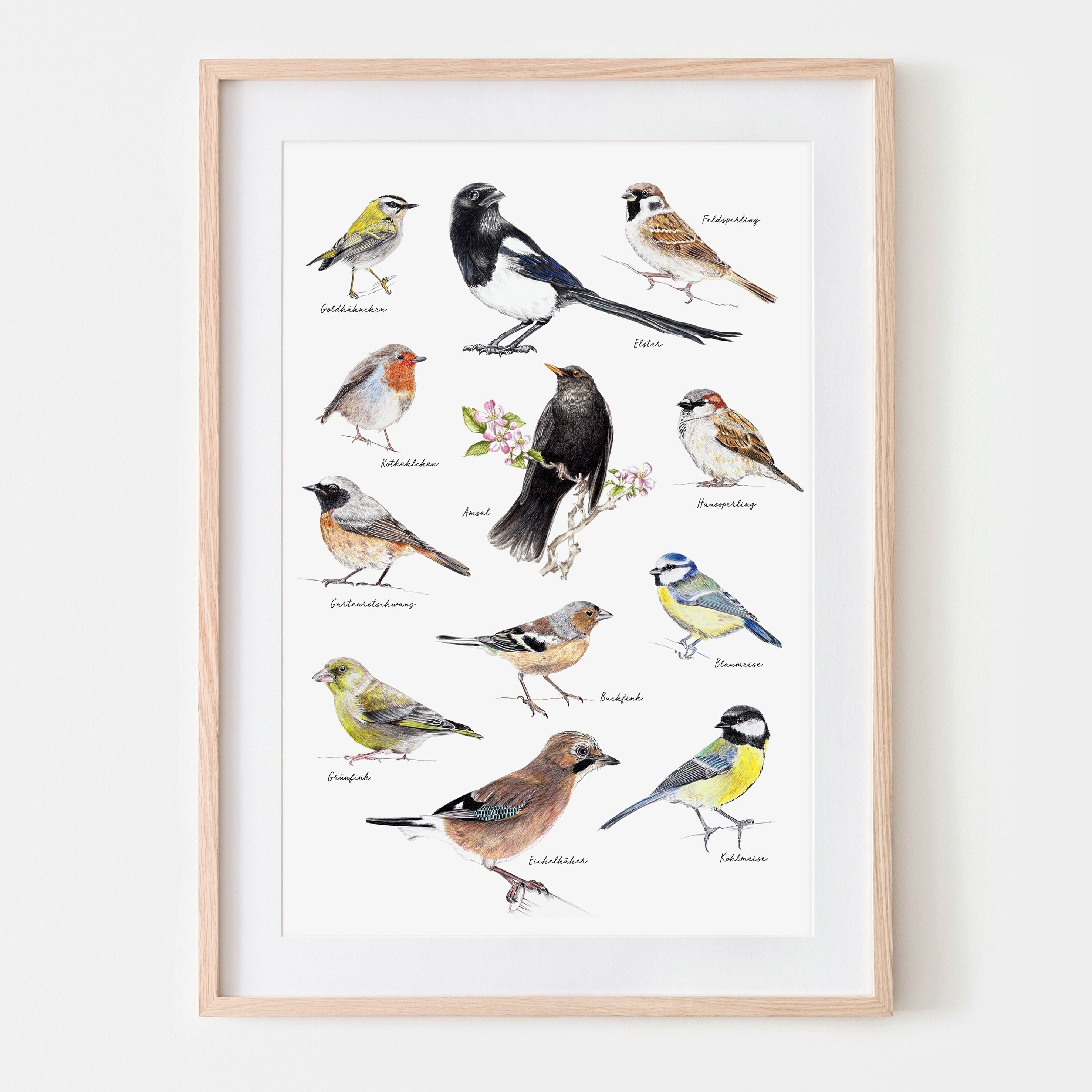This is a full-color photograph showcasing a framed collection of twelve different types of birds. The vertically rectangular image is positioned against a white background with a hint of shadow along its far right side, suggesting it was taken indoors. The frame is simple and wooden with an additional off-white inner frame that surrounds a white backdrop on which the birds are displayed. Each bird is distinctly labeled with its scientific name, though the text is too small to read clearly. The birds, possibly native to North America, exhibit a diversity of colors such as yellow, blue, green, orange, brown, black, pink, tan, beige, and white. They are arranged in a non-linear fashion across the frame, creating a somewhat scattered yet balanced composition.